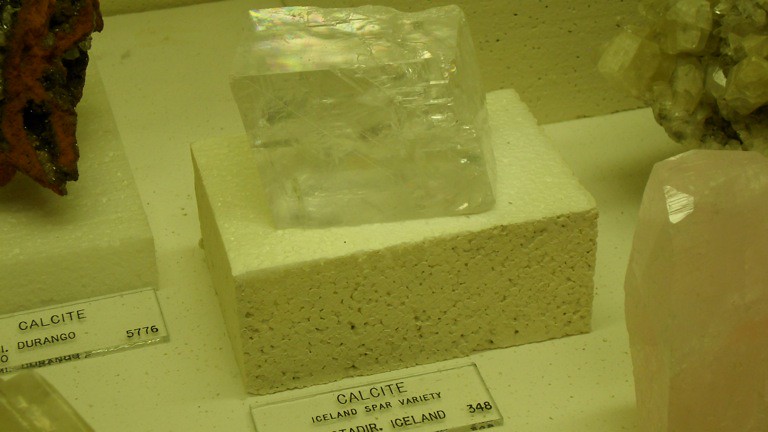The image shows an array of geological specimens, each displayed in a well-organized case with identification tags. The central focus is a yellow Calcite crystal, specifically an Iceland Spar variety, positioned on a yellow display block. This crystal, with its translucent, prismatic structure, boasts sharp angles and an opalescent sheen. Accompanying the display is a transparent label that reads "CALCITE, ICELAND, SPAR VARIETY, NUMBER 348" in capital letters. To the left, there is a reddish and black Calcite crystal from Durango, labeled "CALCITE, DURANGO, NUMBER 5776," also on its own display. Additionally, to the far right, there are two more Calcite crystals without visible labels. The overall lighting is dim, adding a subtle ambiance to the scene, but making it slightly challenging to discern the details of the crystals on the right.